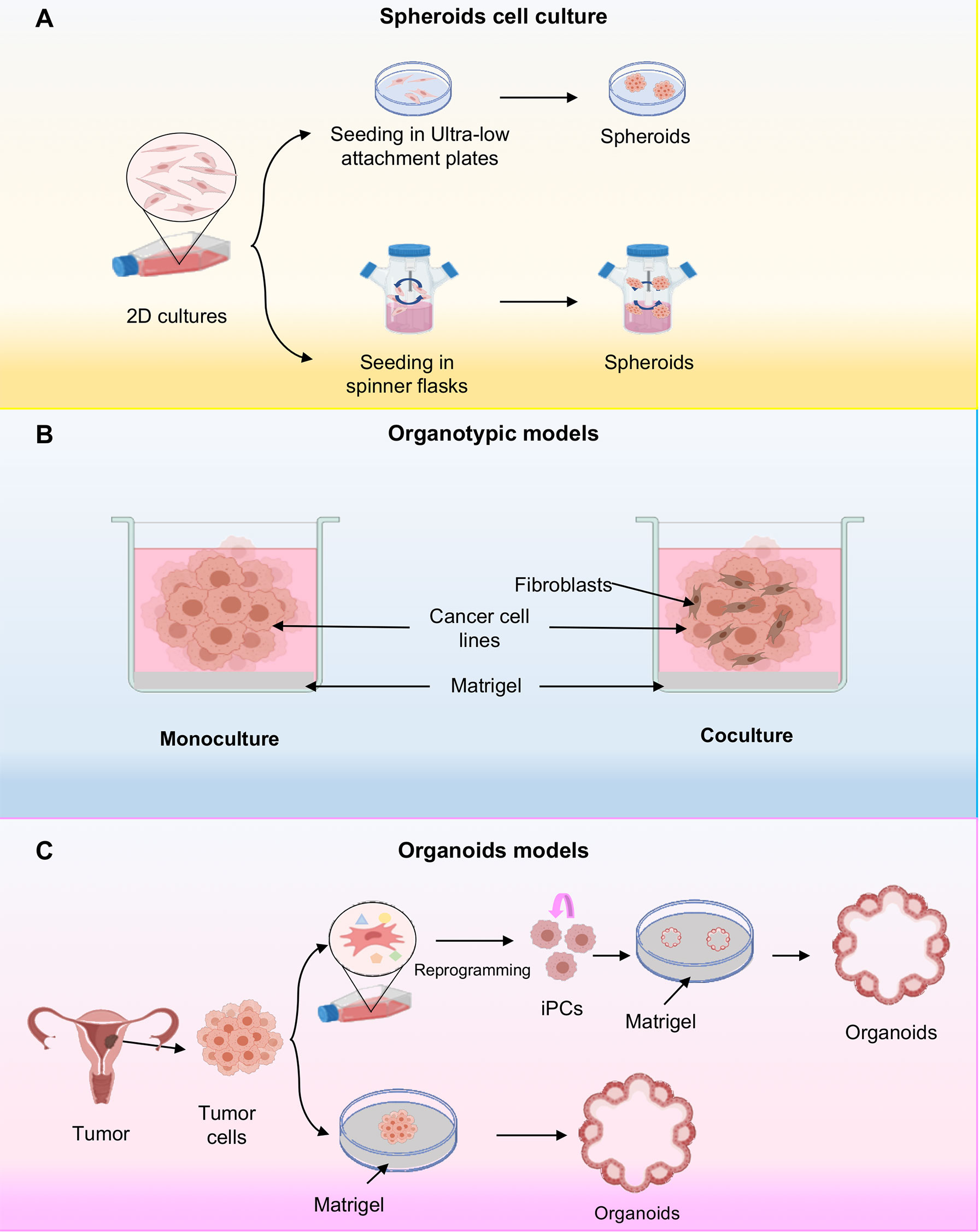The image showcases a detailed scientific poster segmented into three distinct color-coded sections. The top third of the poster, set against a white background, is titled "Spheroid Cell Culture." To the left, under the label "2D Cultures," it displays a sequence of rudimentary drawings and images: a Petri dish with pink spots titled "Seeding and Ultra Low Attachment Plates" leads to another Petri dish with larger pink spots labeled "Spheroids," connected by a black arrow. Below, another set of images show a jar with a blue lid and pink liquid titled "Seeding and Spinner Flask," pointing to a similar jar now labeled "Spheroids."

The middle third, on a blue background, features the title "Organotypic Models." This section splits into two parts: on the left, under "Monoculture," an illustration of a container with pink material connected to labels such as "Fibroblast." On the right, the "Coculture" label accompanies a similar image with additional black lines, also detailed with labels identifying various cellular structures like "Cancer Cell Lines" and "Matrigel."

The bottom third, set against a pink background, is headlined "Organoids Models." It prominently features a diagram of a woman's reproductive system with a highlighted tumor. This illustration points to an enlarged depiction of tumor cells alongside several Petri dishes divided into stages labeled "Reprogramming," "IPCs," "Matrigel," and "Organoids," detailing the progressive cellular transformations within the depicted models.